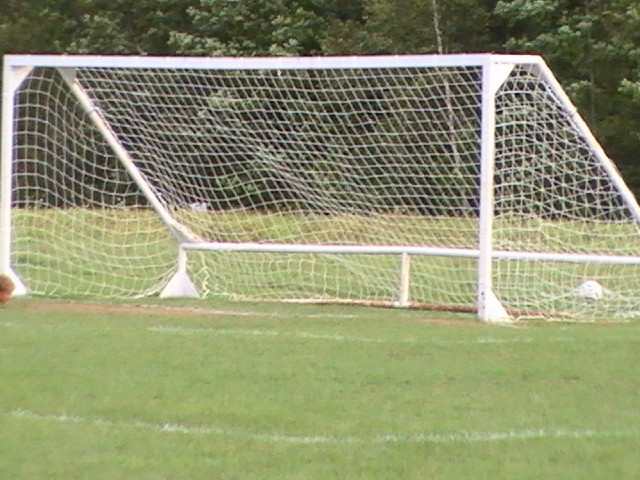In the center of the image, a large white soccer goal dominates the scene with its net hanging at an angle, supported by sturdy white frame posts. The net appears worn in some spots, with patches of dirt peeking through where the grass has been eroded, likely from frequent goalie activity. Nestled behind the goal, a soccer field stretches out with its neatly cut, medium-green grass marked by crisp white chalk lines delineating different sections of the field. In contrast, the background reveals a slightly taller, lighter green grassy area, giving way to a dense backdrop of darker green trees and bushes. Predominantly green and white, the image captures a serene yet actively-used sports environment, possibly even hinting at a soccer ball lodged in the back of the goal net.